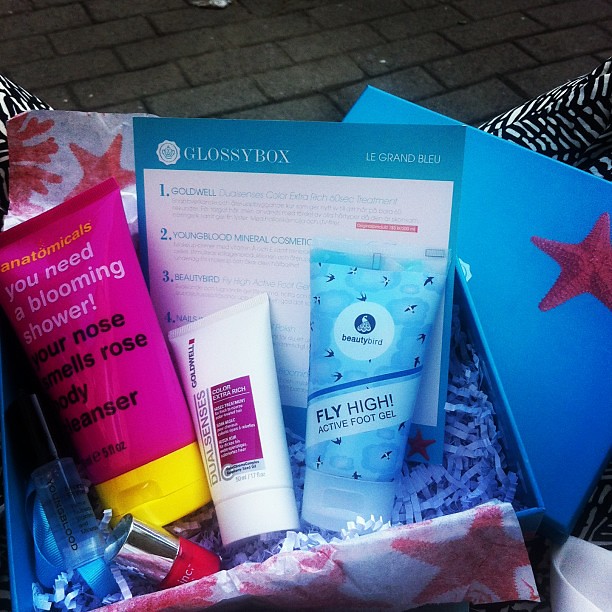The image features an open beauty subscription box, identified as a "Glossy Box," set against a gray brick tile background. The box itself contains various cosmetic products arranged on a bed of blue shredded paper.

On the left side of the box, there's a pink squeeze tube with a yellow cap, labeled "Anatomicals: You Need a Blooming Shower, Your Nose Smells Rose, Body Cleanser." Next to it, positioned toward the base of the box, is a small red nail polish container.

In the middle section of the box, a white tube with a burgundy square in the center sits prominently, though the text on the packaging is too small to read clearly.

To the right of the white tube, a blue-packaged product is visible, identified as "Beauty Bird Fly High Active Foot Gel." Nearby, there's a smaller clear bottle with a black lid.

The box also contains a postcard prominently featuring the words "Glossy Box." The details on the card include further text and numbered lists of cosmetic brands, such as Goldwell, Youngblood Mineral Cosmetic, Beauty Bird, and Nails. Decorative elements like starfish designs are found on the lip and interior of the box, adding to its aesthetic appeal.

Overall, this curated selection of beauty products is presented neatly within a stylish blue box, evoking a sense of thoughtful luxury and attention to detail.